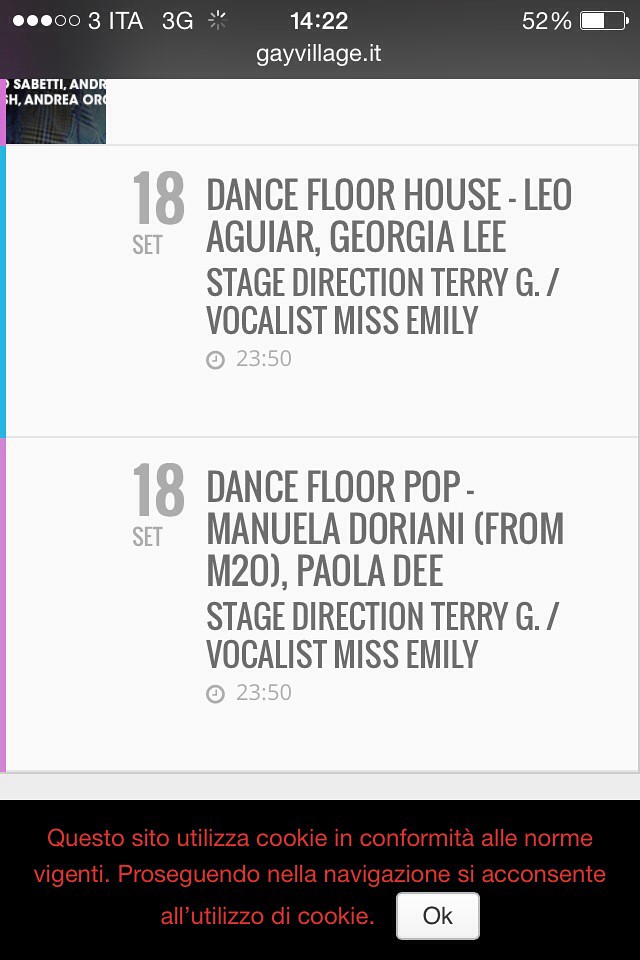The image depicts a detailed screenshot of a phone screen, displaying a schedule for an event titled "Gay Village," with text in Italian. The screen, dated in a 24-hour format at 14:22 with a battery life of 52%, lists two musical sets. The first set, labeled as "Dance Floor House," features performances by Leo Aguirre and Georgia Lee, with stage direction by Terry G and vocals by Miss Emily at 23:50. Immediately following is another set, labeled "Dance Floor Pop," which includes performances by Manuela Dorian and Paola D, again with stage direction by Terry G and vocals by Miss Emily at 23:50. The bottom of the screen contains red text in a different language regarding a cookie policy, with an acceptance option indicated by an "OK" button. The entire image is primarily black and white aside from the red text of the cookie policy.